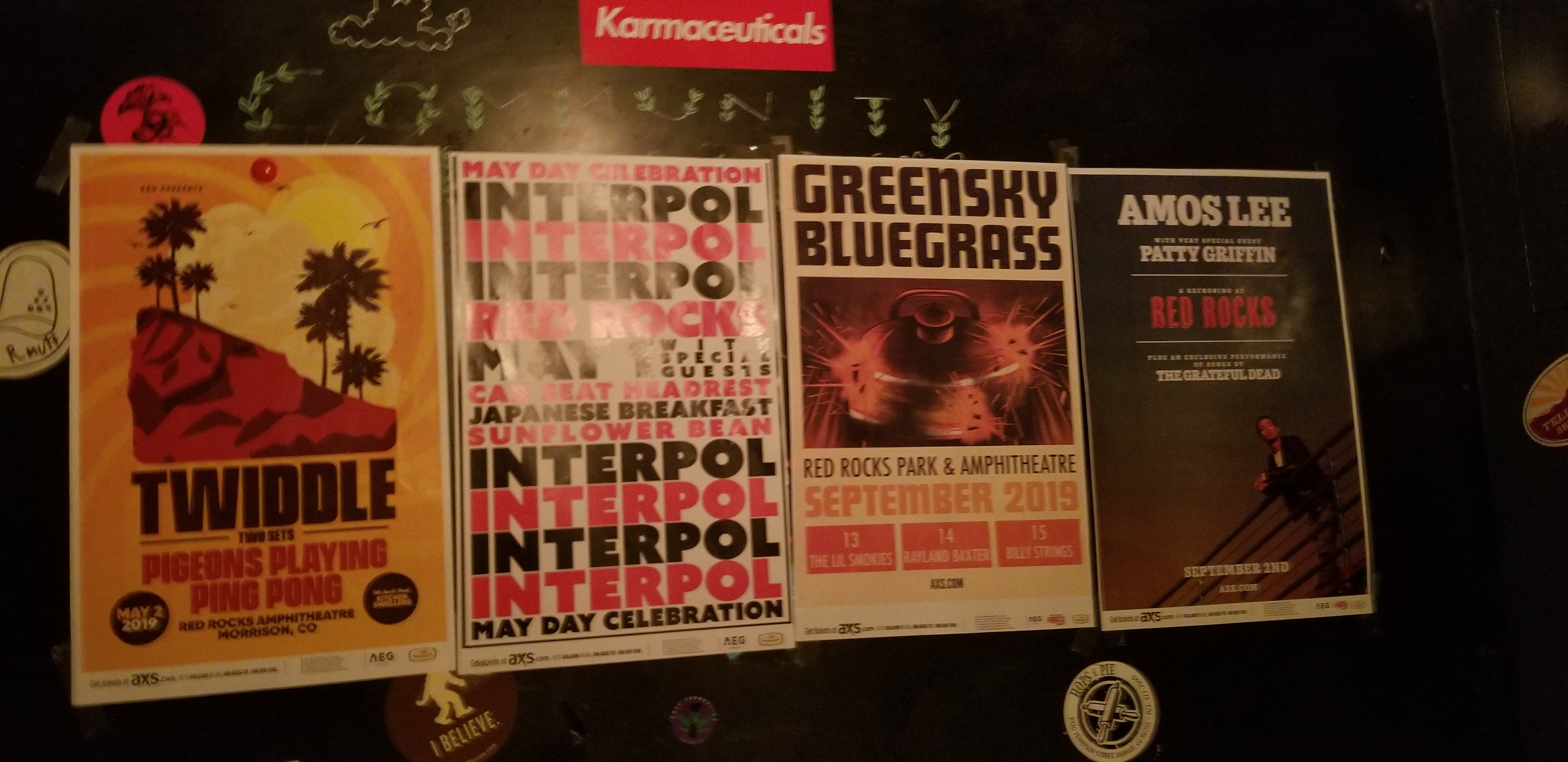The image presents four distinct posters set against a deep black background, topped with a red banner reading "Karmaceuticals." Each poster provides information about different events and artists:

1. The first poster on the far left features an island with palm trees under a yellow sun, set against an orange background. The names "Twiddle" and "Pigeons Playing Ping Pong" are written in brown letters at the bottom.
2. The second poster shows a white background with alternating text colors of brown and red, detailing a "May Day Celebration" and featuring the band "Interpol."
3. The third poster, also on a white background, lists "Green Sky Bluegrass" with the event "Red Rocks Park and Amphitheatre, September 2019" emphasized in bright yellow. Below, three small orange boxes display the dates: 13th, 14th, and 15th.
4. The fourth poster displays a black-coated man leaning over a railing on a deck under a dark brown sky. It reads, "Amos Lee, Patty Griffin" in white letters, with "Red Rocks" highlighted in red.

Overall, these posters collectively announce various musical events with detailed artistic elements, unified under the promotional banner "Karmaceuticals."